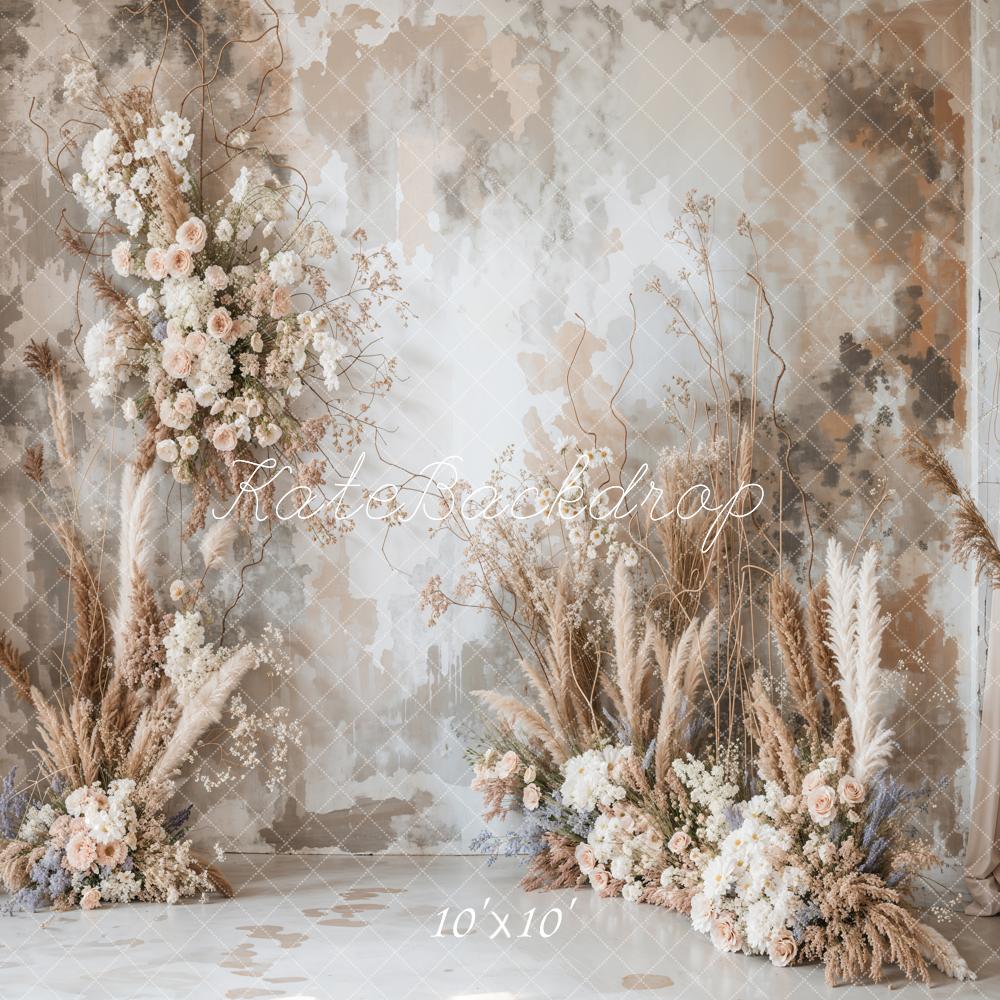The image presents a soft-colored and neutral-toned backdrop titled "Kate Backdrop" in cursive white text across the center and marked "10 feet by 10 feet" in white text at the bottom. The backdrop is designed for photographs and features abstract diagonal patterns with hues of peach, white, soft gray, light brown, and pale pink. It showcases several flower arrangements with light-colored flowers, including pale pink, white, and light blue flowers, interspersed with fall-colored leaves and long, soft plumes resembling wheat sheaths. These floral arrangements are positioned strategically with two on the right side, two on the left, and some seemingly hanging from the ceiling. The backdrop also features a subtle diamond grid pattern made of thin white lines that overlay the entire image, adding texture without overwhelming the serene composition. There is space in the middle, likely intended for individuals to pose, with the left side of the backdrop showing flowers and sheaths of wheat rising from the floor and climbing upward.